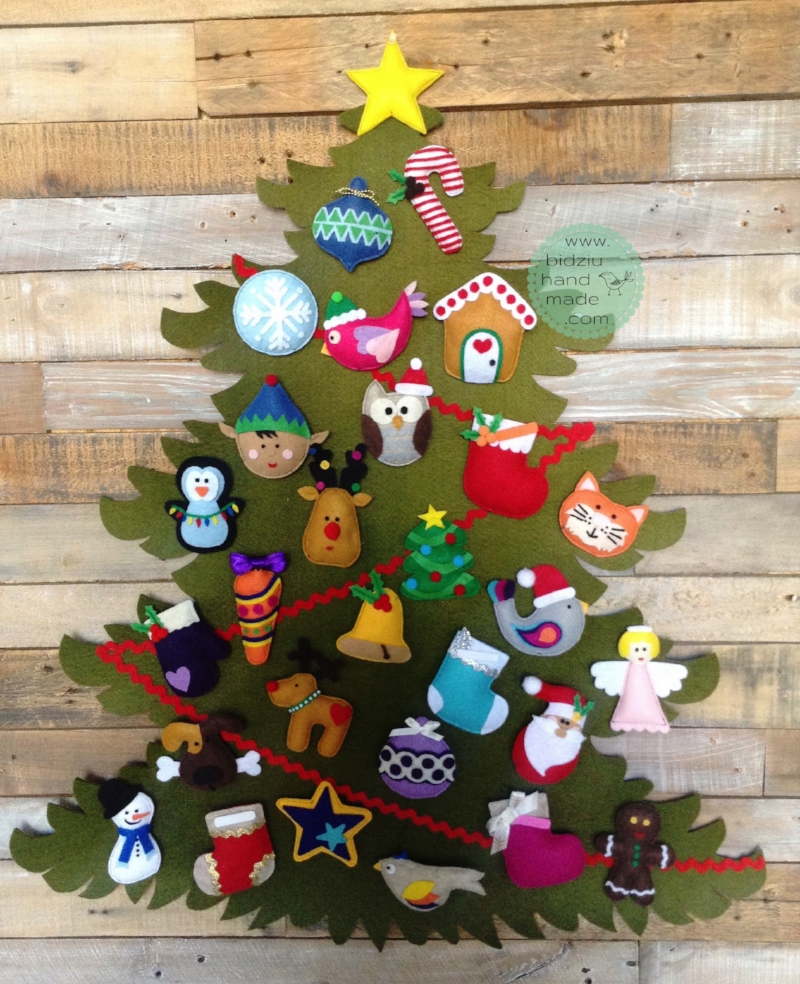This image features a vibrant arts and crafts project showcasing a large, homemade felt Christmas tree displayed against a wood plank background. At the very top of the tree, a gold star gleams prominently. The tree is adorned with a variety of felt ornaments, likely attached with Velcro, creating a playful and interactive design intended for kids. Ornaments include familiar Christmas icons such as candy canes, birds, owls, reindeer, penguins, a bell, a red stocking, a Santa Claus, a gingerbread cookie, a snowman, mittens, a dog with a bone in its mouth, a cat, an angel, an elf, a Christmas tree, and additional stars. There are also less conventional ornaments like a gingerbread house, a snowflake, and a ribbon zigzagging across the tree. This charming, handcrafted piece doesn’t just capture the festive spirit with its diverse ornaments, but also includes a small detail of a website, "www.bidzohandmade.com," enhancing its authenticity and handmade charm.